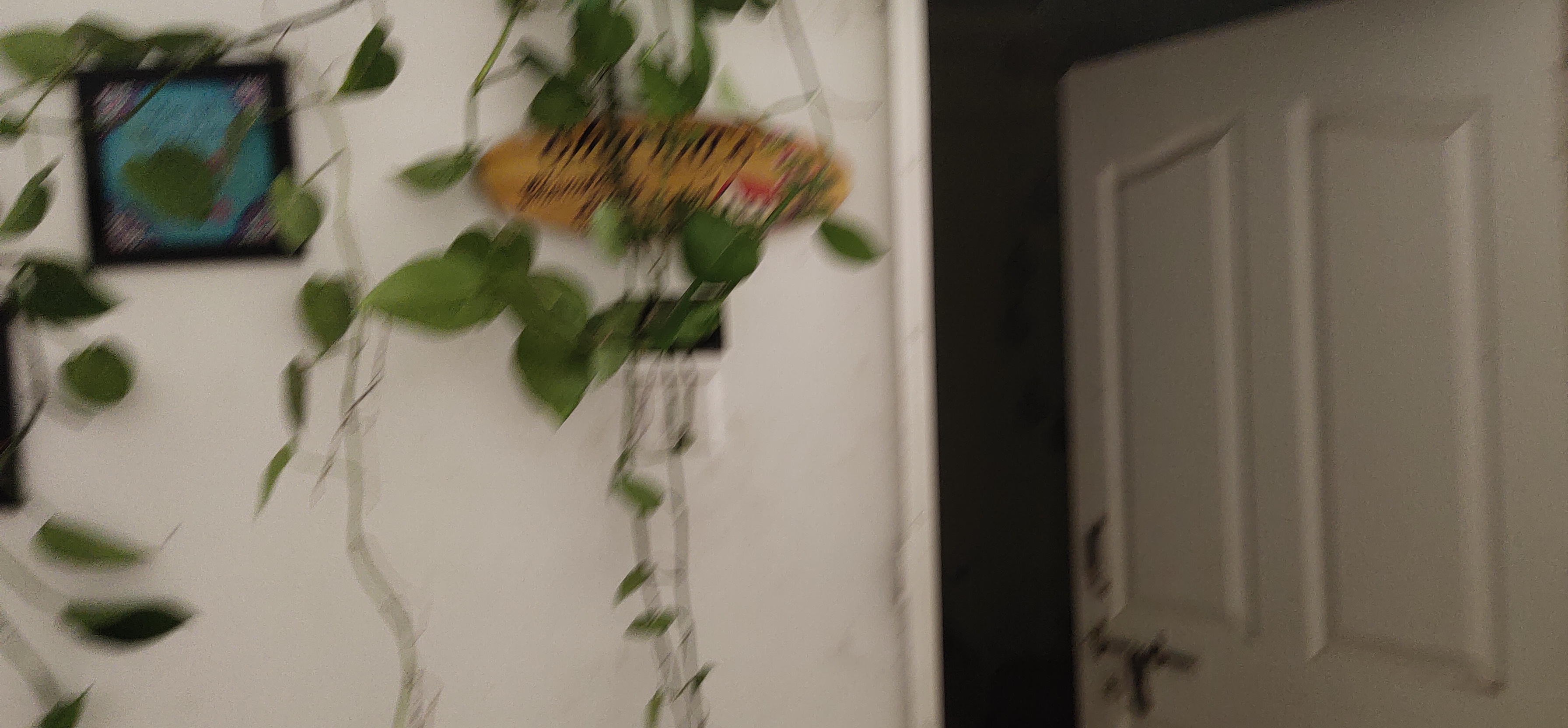The image captures an interior space of a house, featuring a slightly ajar white wooden door. The door is equipped with a cylindrical latch that can be slotted into a hook to secure it. The surrounding wall is also made of white wood, creating a cohesive aesthetic. Adorning the wall is a picture framed by lush vines that add a touch of nature to the scene. The room beyond the door appears darker, emphasizing the contrast between it and the well-lit main area of the image.